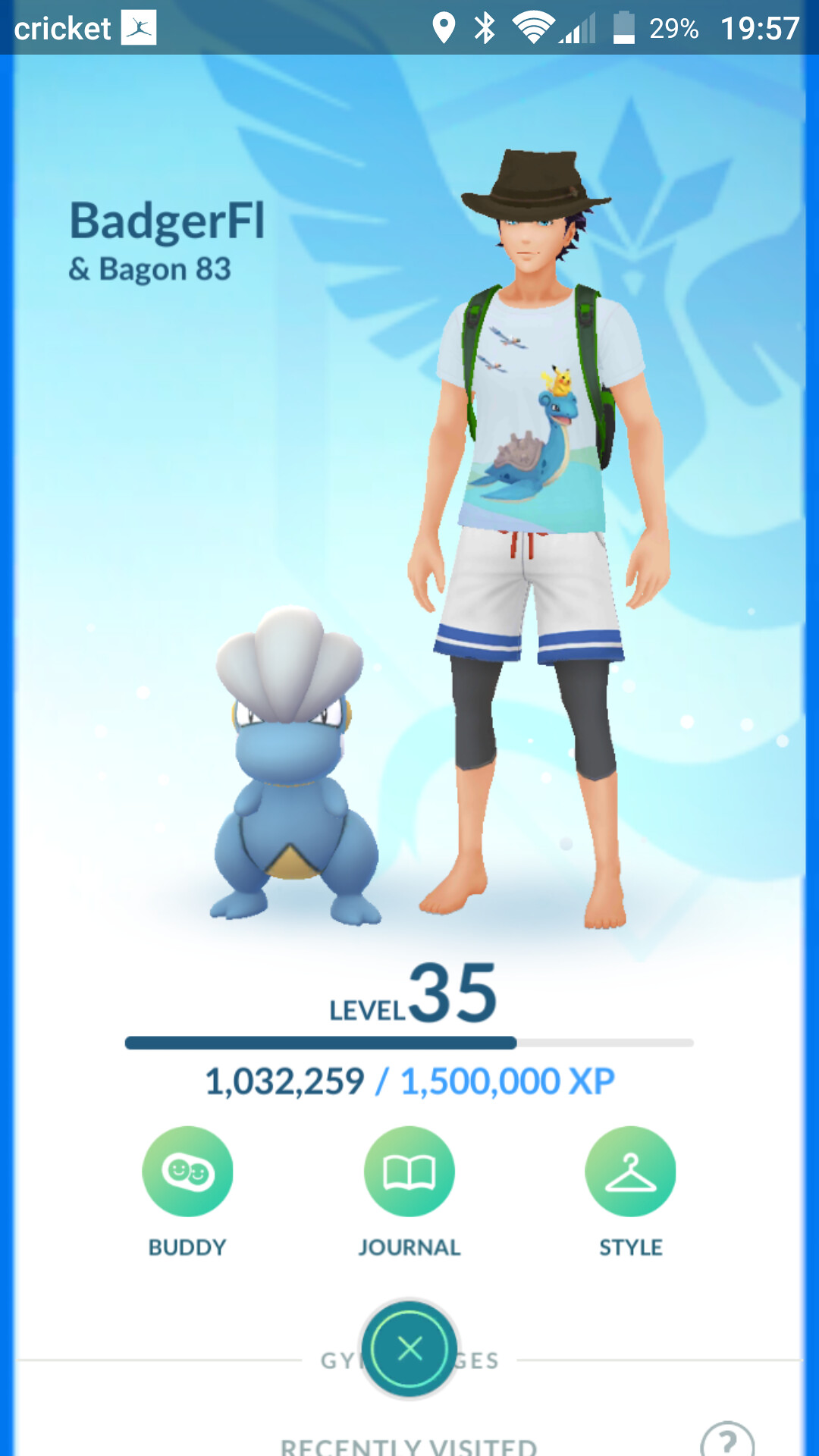This image is a detailed screenshot taken from a mobile device, likely an Android phone, as indicated by the interface elements. At the top of the screen, indicators show the internet connection status, a 29% battery life, and the time, 7:57 PM, with the word "Cricket" in the upper left-hand corner. The center of the screenshot prominently features an animated scene with a male character possessing dark hair and wearing a black hat with a thick brim, a white t-shirt adorned with a cat, a dragon, and two birds, a green backpack, white and blue striped shorts over black leggings. To the left of this character is a small blue dragon-like creature. Adjacent to the characters, text in blue reads "Badger F.I. and Bagan 83." Below this text, the level is indicated as "35," with an experience points bar showing 1,032,259 out of 1,500,000 XP. The bottom section of the screenshot features four icons labeled "Buddy," "Journal," "Style," and an 'X' button for closing the app. The vibrant color palette includes shades of blue, green, yellow, and more, enriching the visual composition of the image.